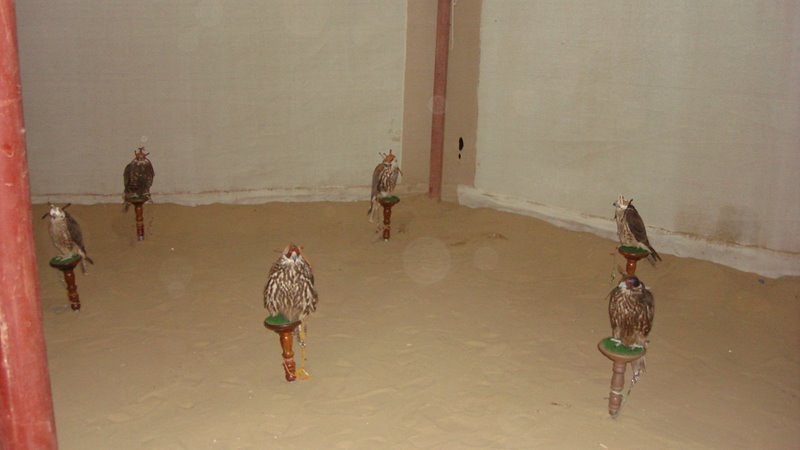The photograph depicts a low-resolution, colour image of a room with a tan floor and worn white walls accented by a maroon beam and pipeline. In the center of the room, six cylindrical wooden pegs are arranged in a nearly oval shape, each topped with a circular green felt platform. Perched on each platform is a bird, likely eagles or hawks, characterized by their brown feathers, which range in shade from lighter to darker hues. Notably, some birds feature red feathered caps and white feathers around their heads. The back corners of the room house rucked canvas, suggesting a temporary exhibit or display setup. The overall image quality is marred by spots, likely due to a dirty lens, contributing to the poor resolution and lack of sharpness.